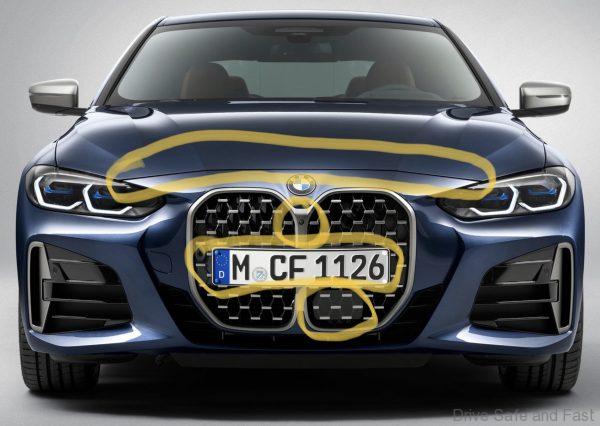This color photograph depicts the front of a sleek, dark blue metallic BMW. The vehicle is positioned against a gray background and has distinctive features highlighted with hand-drawn yellow markings, reminiscent of using a highlighter in a screenshot editing tool. Notable details include the elegant silver-trimmed, dark bluish headlights, and silver side mirrors. The car's grille is divided into two segments resembling an egg crate pattern in silver and black, with two black air inlets featuring slots on the left and right sides. The European-style license plate reads "MCF 1126" in black text on a white background. Several areas on the car are circled, such as the seam at the front of the hood lid, a detail below the badge, the license plate, and a section of the grille at the bottom right. The image also contains a subtle watermark in the bottom right corner with the words "drive safe and fast." The interior, slightly visible through the windshield, appears to feature leather seats. This detailed and annotated image suggests it might be taken from a blog or automotive website.